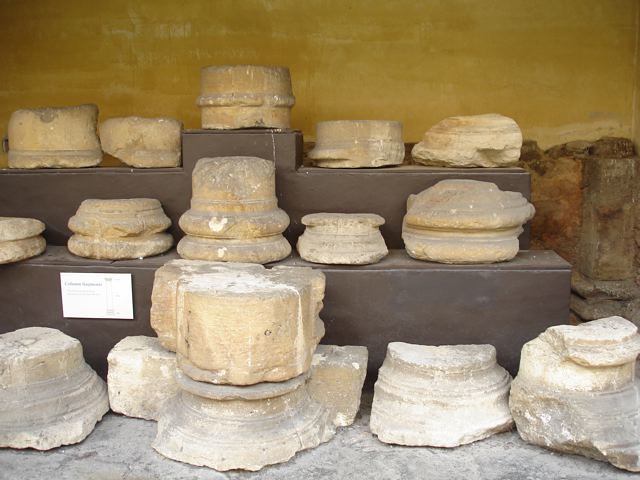The image features a display of archaeological objects, likely parts of old stone columns, arranged on three shelves and the ground in the foreground. The backdrop is a yellowish-brown wall, transitioning to a brown color near the bottom. The two central shelves, likely wooden and brownish in color, hold these relics. The top shelf has five objects, including a central pedestal displaying a round artifact. The next shelf below also houses five rounded objects. The bottom shelf and the objects on it are white, adding a contrasting element to the scene. To the left on the bottom shelf, there's a white placard, typical of museum displays, though the lettering is unreadable from this distance. These stone relics vary in shape—some are round, half-circles, or long like bricks—and many feature distinguishing ridges and lines, indicative of their historical and architectural significance.